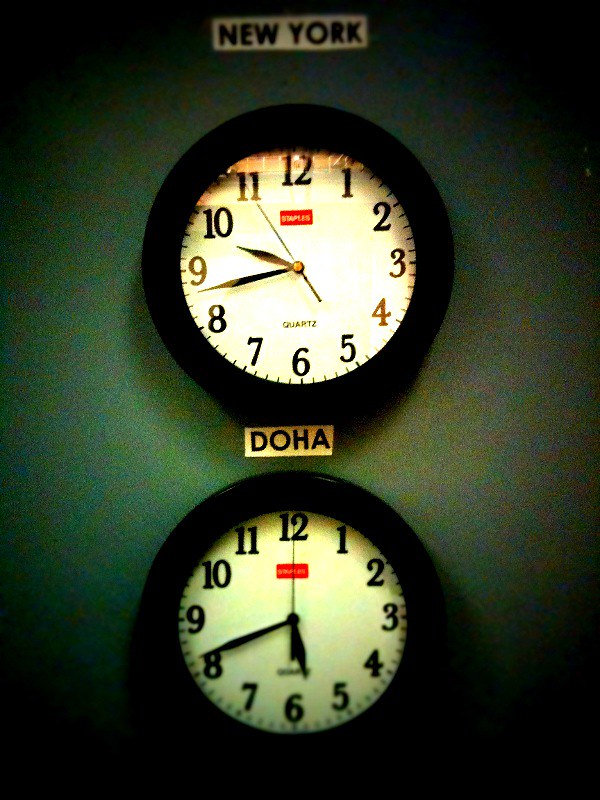The image features a predominantly gray background, which appears to take on a slight greenish hue due to the image's darkness and possible camera ISO effects, manifesting as blue and yellow speckles in the darker areas. The corners of the photograph are entirely black, adding a vignette effect. Centrally situated are two identical clocks, one positioned above the other. The upper clock is labeled "New York" with a white-bordered black print, while the lower one is labeled "Doha" (spelled D-O-H-A). Both clocks feature white faces, each adorned with a red block displaying the word "Staples" in white letters and the word "Quartz" in black lettering. The clocks have numerals 1 through 12 with hash marks in between each number. The time displayed on the New York clock is 9:43, whereas the Doha clock shows 5:41.